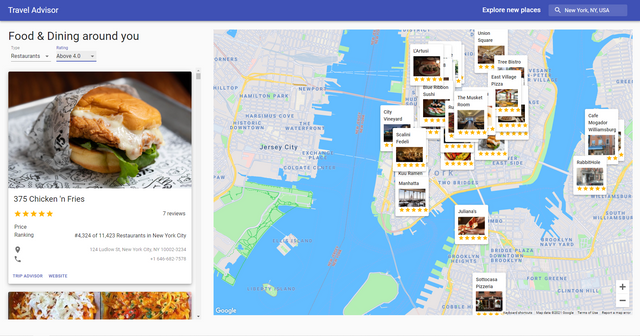A screen capture from the Travel Advisor website displays a well-organized interface within a purplish-blue bar header. The left side of the bar reads "Travel Advisor" in white letters, while the right side proclaims "Explore New Places" in the same font color. Adjacent to the right, there is a search bar, with the placeholder text "New York, New York, USA" in white, next to a magnifying glass icon.

On the left side of the screen, a vertical banner is labeled at the top in black text, "Food and Dining Around You." The filter options are set to display restaurants with ratings above 4.0. Below this banner is an image of a chicken sandwich perched on white and gray tissue paper. The label underneath identifies the restaurant as "375 Chicken and Fries," featuring a five-star rating and additional details in small black text.

Directly under the chicken sandwich image, the upper portions of two more images are visible, seemingly depicting pizzas. The main portion on the right side features a detailed map of lower Manhattan, with the shoreline of Jersey across the Hudson River and the shores of Queens and Brooklyn across the East River. Various images with white backgrounds are scattered across the map, each labeled and accompanied by a star rating, indicating popular spots and eateries in the depicted areas.